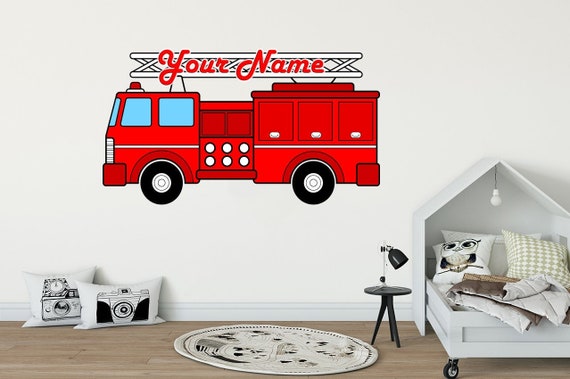The image depicts an intricately designed bedroom centered around a red fire truck decal with black wheels and blue windows on a white wall. The fire truck features a white ladder on top, above which, in red cursive letters, it says "your name," indicating customization options. The bedroom has a light hardwood floor adorned with a black and white rug, accompanied by two black and white pillows on the left featuring camera and clock images. To the right stands a small black table with a black desk lamp. The highlight of the room is a unique fold-up bed that resembles a house, currently pulled down, with a selection of pillows, including one with an owl and a green and white checked one. Above the bed hangs a single light bulb, emphasizing the cozy yet whimsical atmosphere of the space.